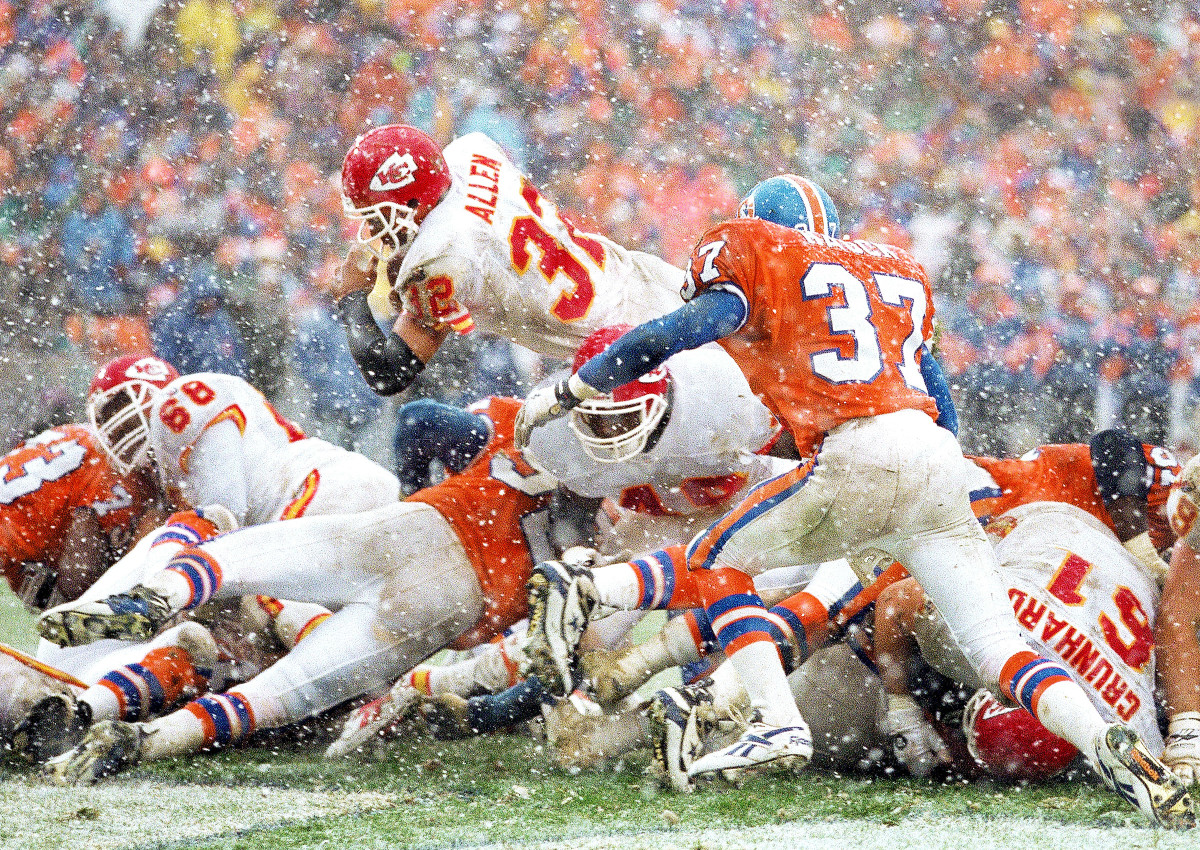In this live-action photograph of an NFL football game, a tense moment is captured as a Kansas City Chiefs player, identified by the name "Allen" on his back, dives over a pile of approximately a dozen players. The scene is set on a snow-covered turf field, intensifying the drama as white flecks of snow or rain fall from the overcast sky. Allen, wearing a red helmet and a white jersey with red lettering, is mid-air, seemingly holding the ball while evading players from the opposing team. The Denver Broncos, distinguished by their dark orange jerseys with blue and white accents, contending with white jerseys and blue helmets, are arrayed in the chaotic pile beneath him. In the blurred background, a packed stadium brimming with spectators can be seen, most donning orange apparel with some in blue, collectively bracing against the cold in heavy coats. The sense of motion and energy in this wintry game day snapshot is palpable.